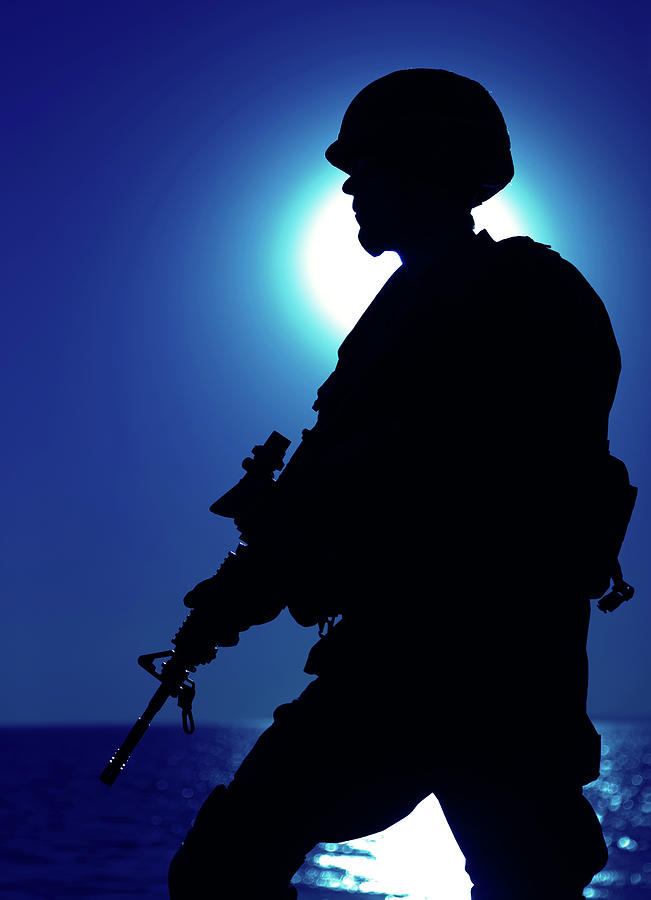In the image, a soldier's silhouette stands prominently against a dark blue sky illuminated by the moon. The moonlight creates a striking reflection on the water below, suggesting the soldier is on a boat or skiff. The infantryman, identified by his helmet with a chin strap, carries a long rifle, possibly an M16 or M4 equipped with a short scope. His stance, with one leg forward, conveys a sense of movement or readiness. The dark, featureless silhouette of his figure due to the backlighting reveals a shallow backpack. The vast expanse of water and sky merge seamlessly on the horizon, with no land in sight, enhancing the solitary, contemplative mood of the scene. The glimmering reflections on the water beneath his legs and around his head underscore the serene yet powerful presence of this lone soldier under the night's embrace.